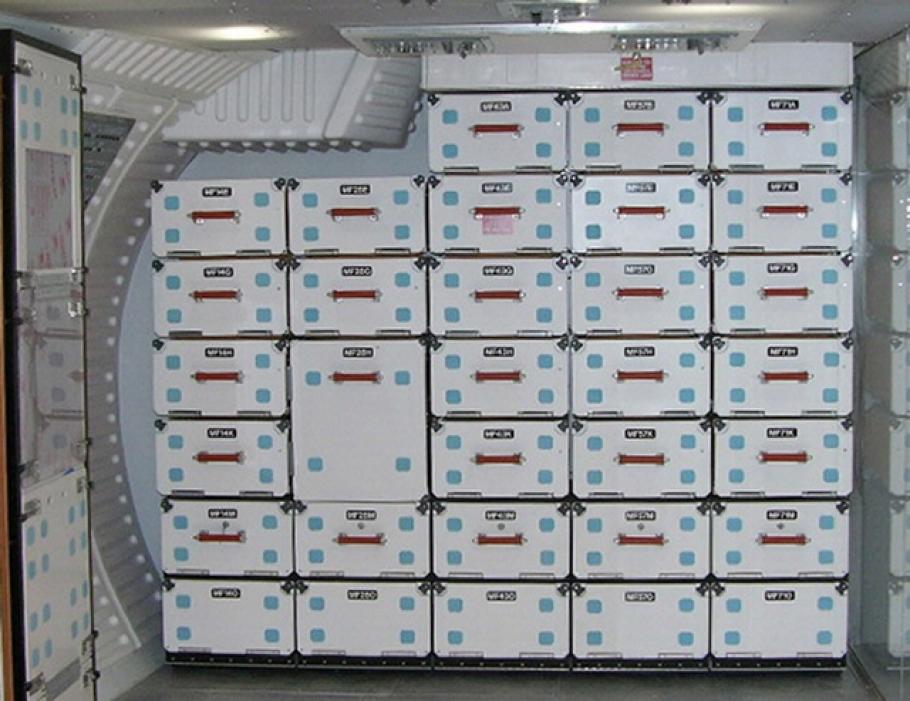The image features a meticulously organized array of drawers, primarily made of white enamel or metal, evocative of a futuristic or spaceship-like environment. The drawers are stacked in multiple columns and rows, creating a sense of symmetry and order. On the left side, there appears to be a set of six drawers partially concealed behind a wall, with a visible section of five drawers in front. In the center, there is a peculiar arrangement where one column has a combination of two smaller drawers merging into one, surrounded by columns containing seven drawers each. 

Interestingly, while most of the drawers are equipped with distinctive red handles, the lower drawers lack these and instead feature small blue squares on either side. The backdrop includes a light blue wall, accentuated by white curved elements with intricate grooves, contributing to the high-tech ambiance. A metal structure is noticeable on the ceiling, adding to the industrial aesthetic. There are hints of additional drawers to the left and possibly to the right, though their details are not as clearly depicted, possibly due to reflections or obstructions.